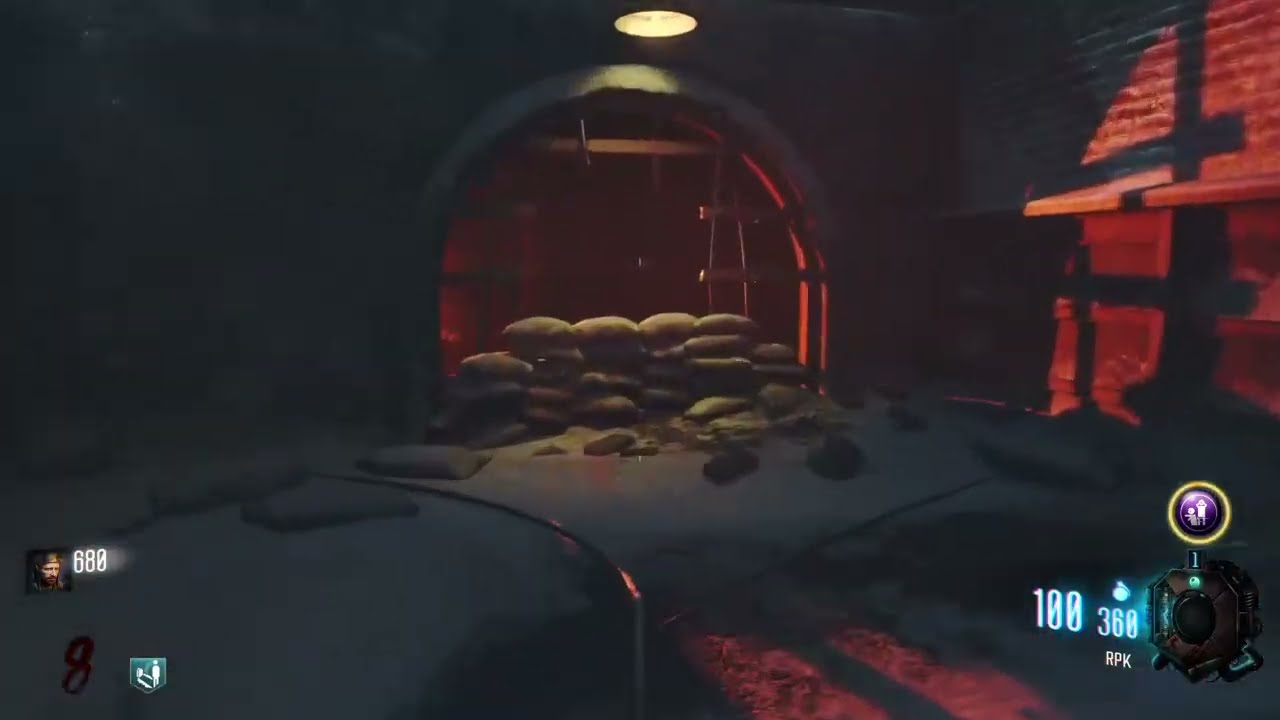The image depicts a dark scene from a video game, likely set indoors in a dungeon or cave-like environment. The majority of the screen is enveloped in darkness, save for the central top portion, where a light source illuminates an arched entryway with red, sand-colored walls, sandbags, and broken metal bars. On the right side of the screen, a red brick wall is partially visible, casting shadows that add to the ominous atmosphere. The bottom right corner displays numbers — “100, 360, RPK” alongside a small, mechanical-like icon. Additionally, a small icon of a man is shown on the left with the number “680” next to it. The overall scene is foreboding, suggesting the main character, possibly a young man with a beard, is navigating a perilous and confining environment, potentially a dungeon or a jail cell.